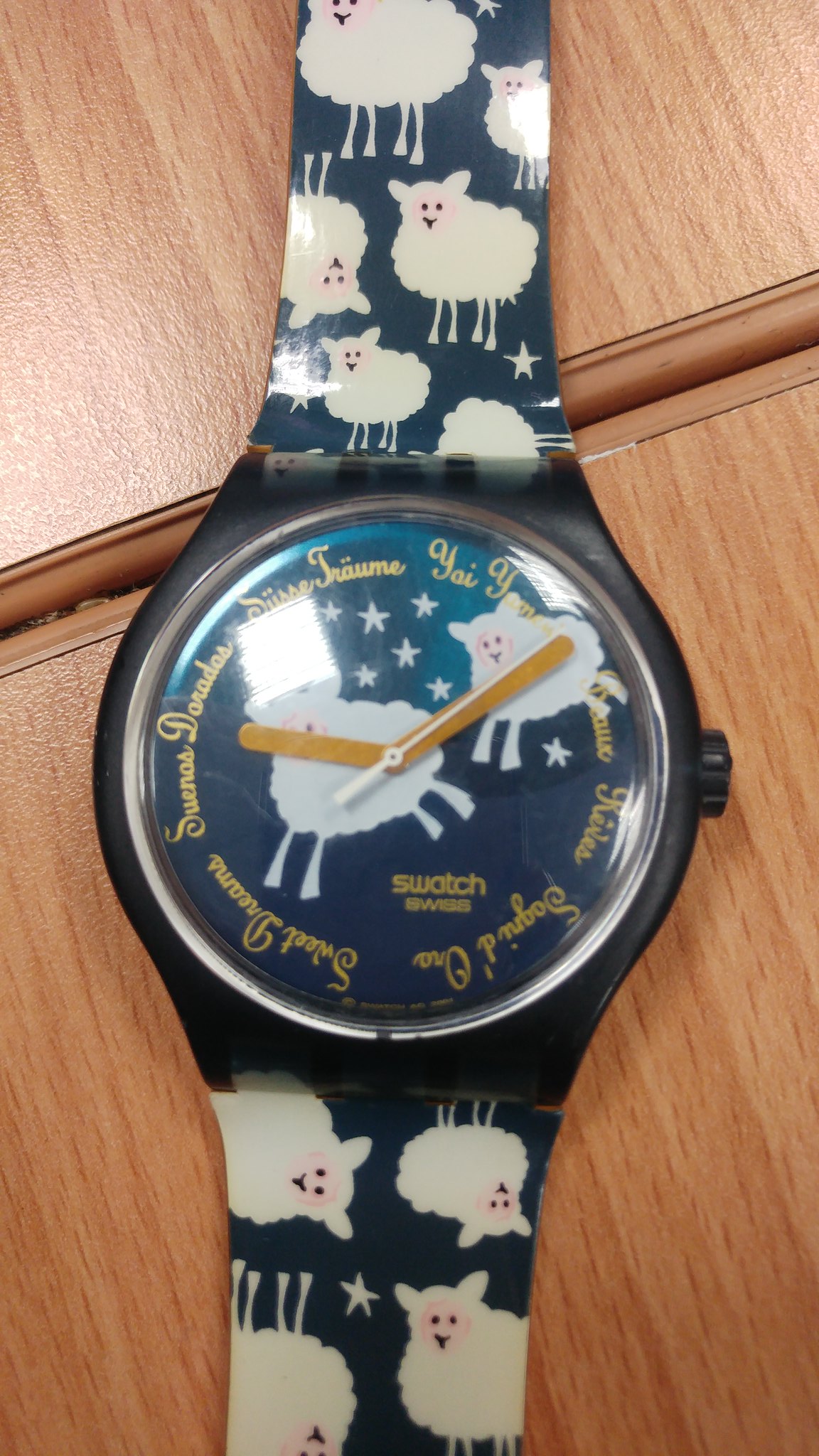This top-down photograph showcases a Swatch wristwatch with a charming sheep theme. The watch, resting on a light tan wood veneer table with darker tan grains, features a dark blue face adorned with two white, fluffy cartoon sheep with pink faces, white legs, ears, and small beady black eyes arranged in a T-shape for their noses. Encircling the watch face are the words "Sweet Dreams" in multiple languages in golden text. The watch's black or dark blue casing complements its dark blue rubbery or plastic band, which is decorated with a pattern of white cartoon sheep and small white stars. The Swatch logo, along with 'Swiss,' is displayed at the bottom right of the face. The watch currently shows the time as 9:10.